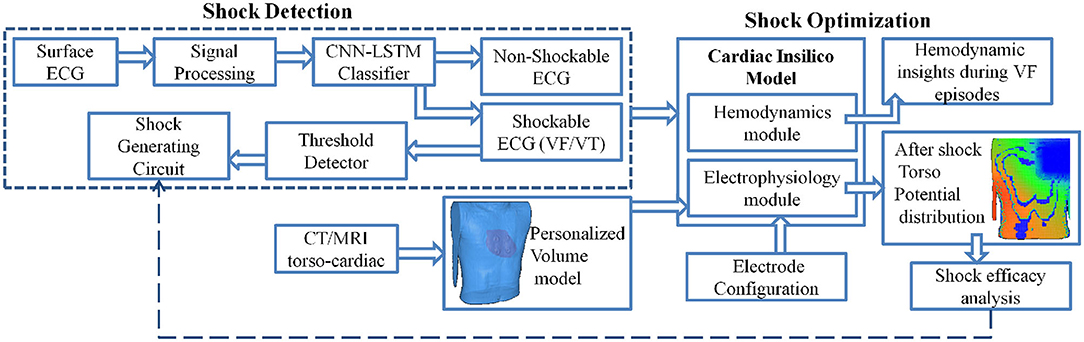The detailed diagram is split into two main sections: Shock Detection on the left and Shock Optimization on the right. 

In the Shock Detection section, the process begins with Surface ECG, followed by Signal Processing. Next in line are CNN, LSTM, and Classifier modules. The pathways then diverge into Non-shockable ECG or Shockable ECG, with further analysis by a Threshold Detector. The process concludes with the Shock Generating Circuit.

The Shock Optimization section includes a Personalized Volume Model involving input data from CT, MRI, Torso, and Cardiac scans. Below this model lies the Cardiac In Silico Model, subdivided into the Hemodynamics Module and the Electrophysiology Module. The Hemodynamics Module provides insights during VF episodes, and the Electrophysiology Module covers aspects such as aftershock torso potential distribution and shock efficacy analysis. 

Together, the diagram illustrates a comprehensive workflow from detecting cardiac shocks to optimizing the delivery and effectiveness of the shock intervention.